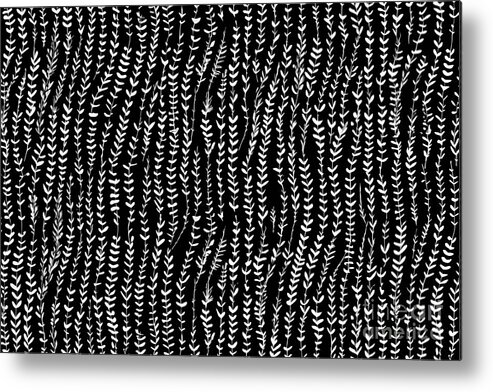The image showcases a sophisticated black-and-white design that appears either hand-painted or expertly printed. Set against a solid black background, the artwork features numerous vertical, wavy white strands, reminiscent of seaweed or fern leaves gently swaying underwater. Each strand is punctuated by small, triangular, heart-shaped elements, resembling leaves or abstract silhouettes of birds, which evoke a sense of natural, fluid movement. This intricate pattern, devoid of any repeating segments, suggests originality and a personal touch, making it suitable as wallpaper, wrapping paper, or a website background. The image, likely a framed piece hanging on a white wall, strikes a balance between simplicity and elegance.